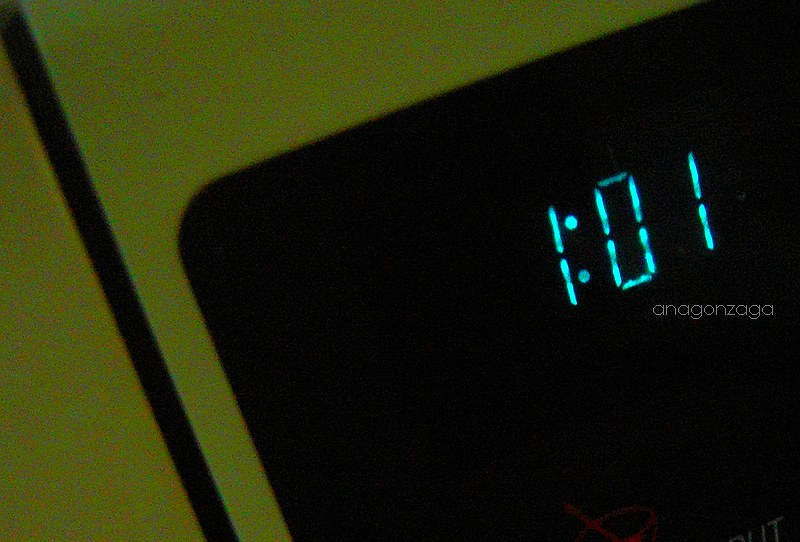The image is a close-up, slightly tilted at a 45-degree angle, of a digital clock on what appears to be a microwave. The clock displays the time as 1:01 in blue LED digits within a black rectangular display. Surrounding this display is a border of greenish or yellowish plastic, with an additional black stripe running diagonally from the upper left to the lower right of the image. To the left of the display, part of a latch corresponding to the microwave door is visible. The photo contains a watermark in all lowercase letters, "ana gonzaga," located beneath the time display. The context is limited to just this close-up view, providing a detailed look at the digital clock's time indication and exterior features.